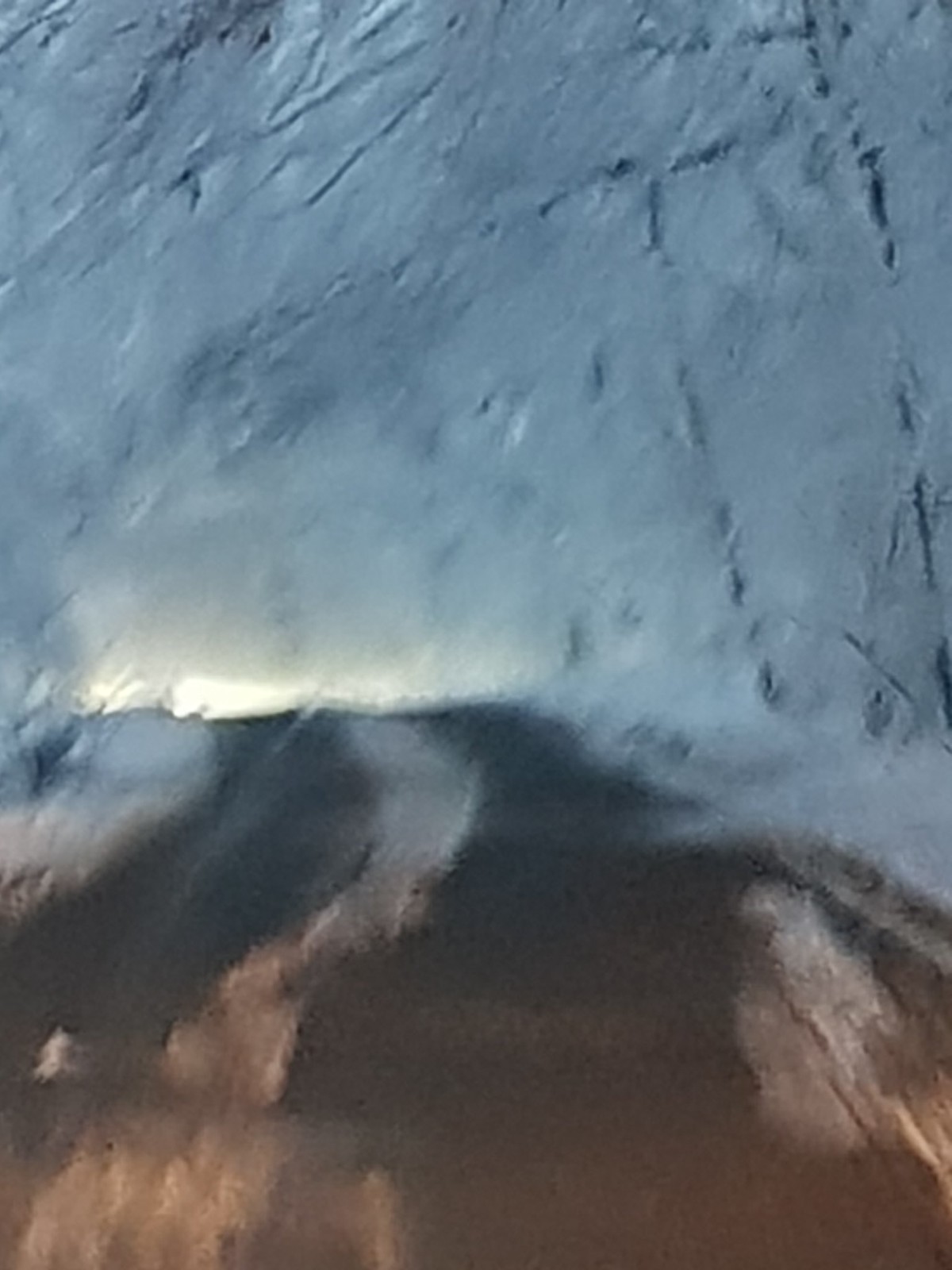The image is quite blurry, depicting what seems to be a mountainous area. The view is down a roadway that has a bluish-gray tint dominating the entire scene. Despite the blur, it appears that the road is brown and possibly covered with snow or debris, suggesting that it is a mountain road. Towards the end of the roadway, there is a visible light, likely the sun, breaking through the haze. Although details are difficult to discern, the image conveys the rugged and rocky terrain of a mountain landscape with a roadway cutting through it.